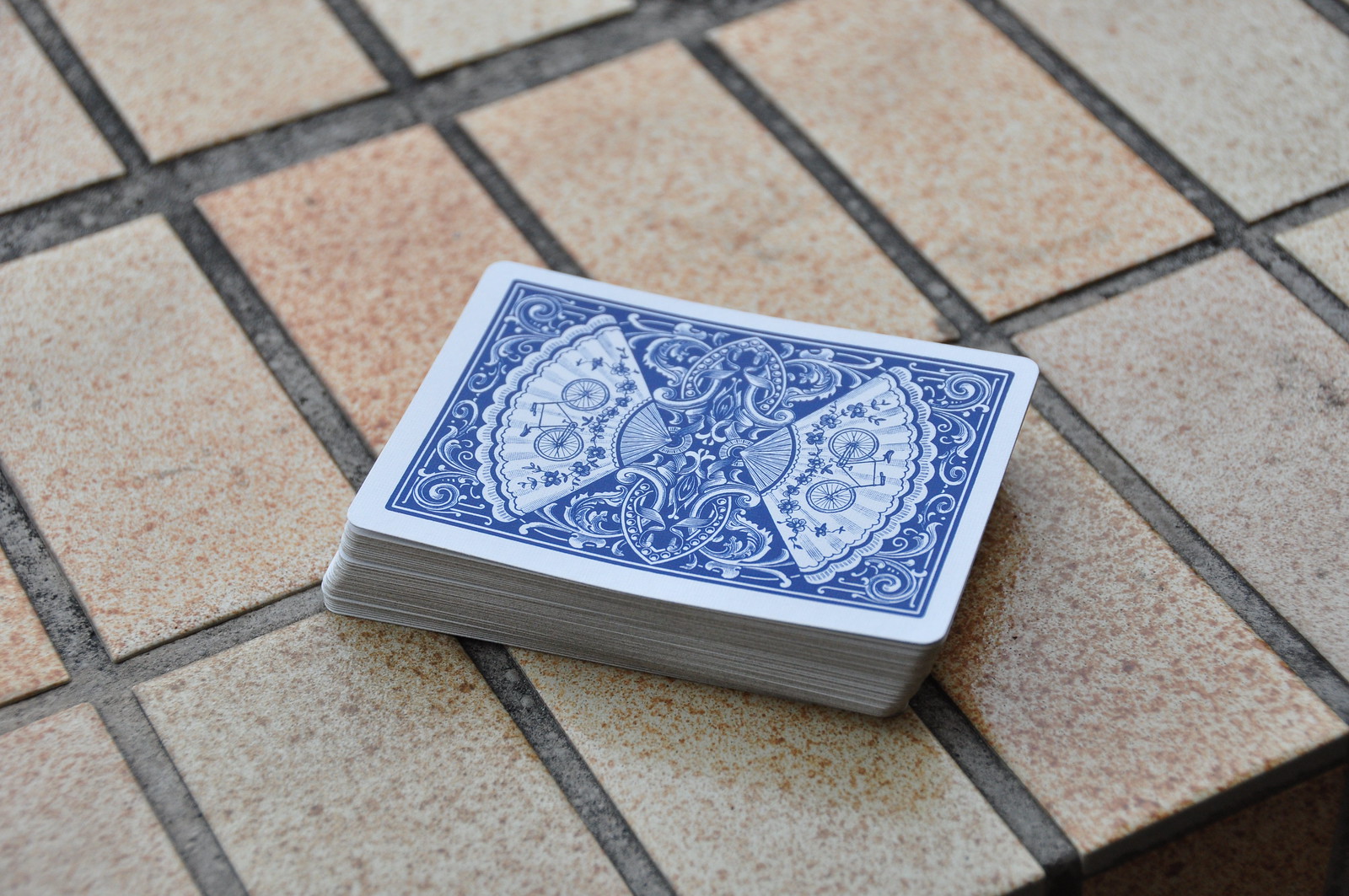This photograph features a diagonally arranged set of fabric or linoleum tiles, predominantly in hues of sandstone that range from light tan to a pinkish shade. The pinkish tiles are subtly speckled with minute gray flecks, adding a textured element to their appearance. The grout lines between the tiles are variations of gray, trending towards charcoal gray.

In the lower right corner of the image, there is a triangular area also in charcoal gray. Positioned centrally in the image, but slightly offset towards the upper left corner, is a diagonal stack of playing cards. The cards are angled from the top left to the lower right of the photograph, featuring white edges and a blue background.

Flanking either side of the card stack are two white fans with scalloped edges, one pointing towards the right side of the image and its mirror counterpart pointing towards the left. Each fan showcases the traditional Bicycle Playing Cards logo, with a blue bicycle design set against a white background.